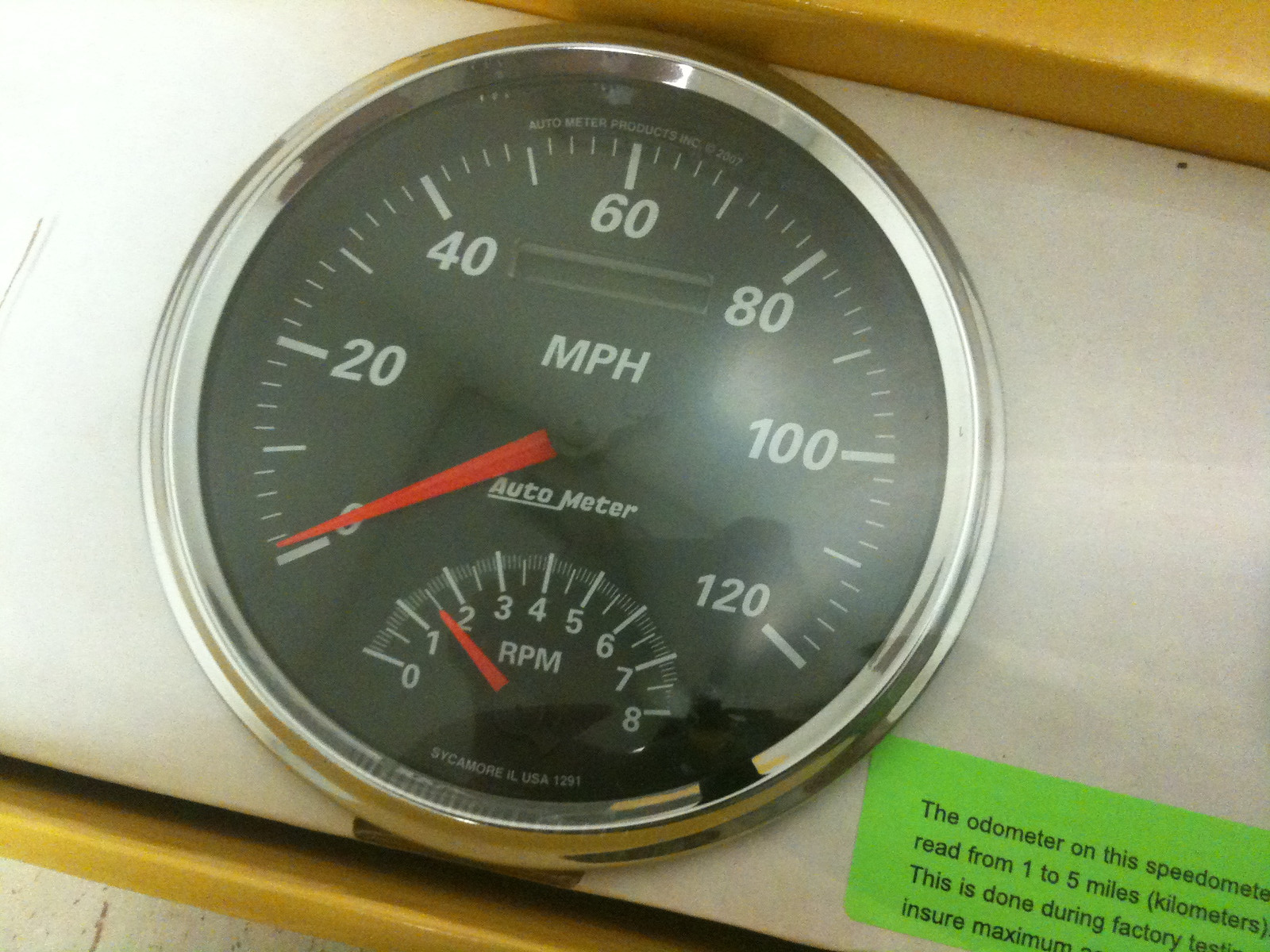The image is an extreme close-up of a vintage speedometer on an old white dashboard. The main dial is black with white numbers and hash marks, with larger hash marks indicating increments of 10 miles per hour, labeled only at every other interval: 20, 40, 60, 80, 100, and 120 mph. At the center of this dial, "MPH" is prominently displayed above the text "auto meter" in white lettering. The red needle on this speedometer hovers just above the zero mark, indicating the vehicle is barely moving. 

Below the speedometer is a smaller half-dial for the RPM, ranging from 0 to 8 with larger hash marks at each number. The RPM dial also includes smaller intermediate hash marks. The red needle on this RPM dial points to the 1.5 mark, further suggesting the vehicle is idling or moving slowly.

Both dials are encased in a round, silver casing. Adjacent to the speedometer, on the right side, is a partially visible blue sticker. The top line reads "The odometer on this speed meter," followed by "read from 1 to 5 miles, kilometers in parentheses." The last two lines of text on the sticker, partially cut off, mention factory testing and ensuring maximum standards.

This detailed image captures the essence of an old-time vehicle's dashboard, highlighting the intricate details and the nostalgic design elements.